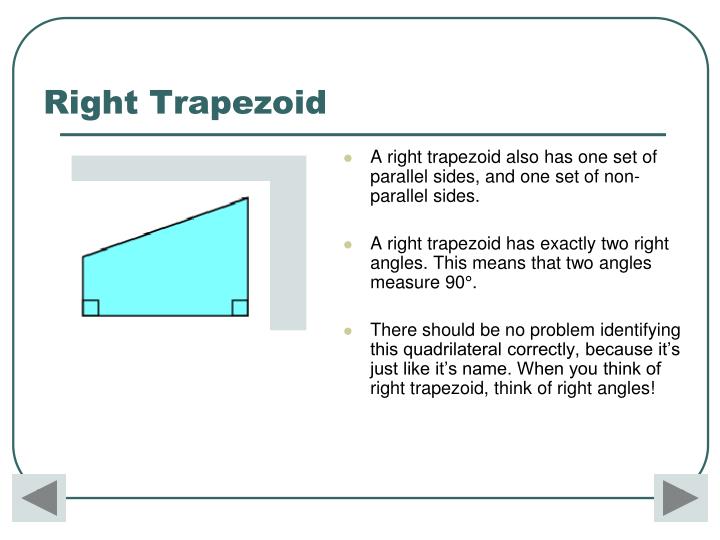This image is an educational slide about right trapezoids. The slide has a rectangular shape with rounded edges and a gray border. The title "Right Trapezoid" is left-aligned at the top in bold, dark gray letters. A horizontal gray line separates the title from the main content.

On the left side of the slide, there is an illustration of a right trapezoid shaded in light blue. This trapezoid has two right angles, one on the left and one on the right, with the right side being higher than the left. The left and right sides are connected by a straight horizontal line at the bottom and a slanted line at the top.

On the right side of the slide, there are three bullet points providing information about right trapezoids:
1. A right trapezoid also has one set of parallel sides and one set of non-parallel sides.
2. A right trapezoid has exactly two right angles. This means that two angles measure 90 degrees.
3. There should be no problem identifying this quadrilateral correctly because it’s just like its name. When you think of a right trapezoid, think of right angles.

The bullet points are gray-colored, and the text is black, all over a solid white background. The entire layout suggests it is part of an interactive presentation, as indicated by left and right arrows at the bottom corners, allowing navigation between slides.